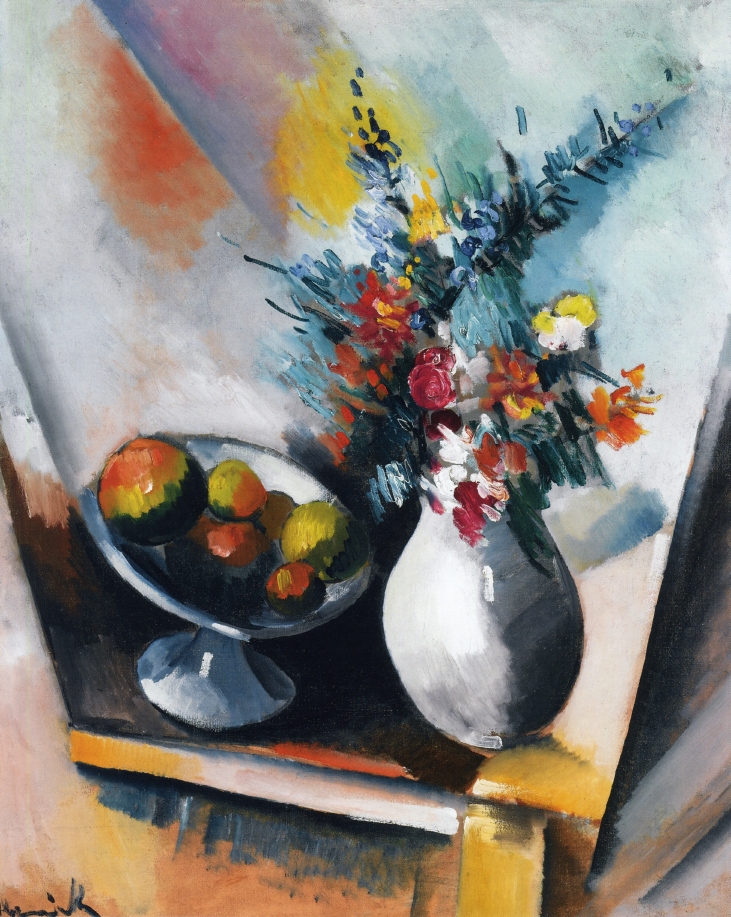This artwork, in the style of a watercolor painting, depicts a painting within a painting set indoors. The central focus is a vase with a bulbous shape, holding vibrant flowers in shades of red, orange, and yellow, accented with green branches. Adjacent to the vase is a black and white pedestal bowl containing five pieces of fruit in various sizes and colors—orange, green, and red. The backdrop of the inner painting features a blend of white, orange, red, and turquoise hues, while dark blue tones dominate the bottom of the painting. The artwork is portrayed on a canvas with a visible frame, suggesting it is displayed on a wooden easel. Additionally, there's an unreadable signature or text situated in the bottom left corner, likely indicating the painter's name. The overall effect is two-dimensional, with the colors creating a bright, vivid presentation that contrasts with the darker elements on the tabletop below the central objects.